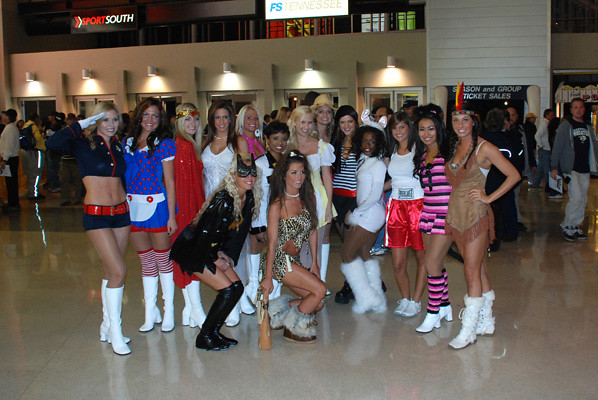The image showcases a group of 14 women, likely cheerleaders or participants in a themed event, posing in front of several ticket booths at a large stadium or convention center. The women, dressed in a variety of costumes ranging from skimpy to slightly longer outfits, include themes such as a Native American, Catwoman, and Wonder Woman, among others. Two of the women are bending down in the front, looking off towards the right, while the rest face the camera. The background features signage such as "Sports South" and "FS Tennessee," illuminated by lights above the ticket booths. Additional text on the right side indicates "Season and Group Ticket Sales." The floor is shiny and tiled, reflecting the overhead lights. Numerous people in the background are lined up and observing the women, contributing to the bustling atmosphere of the event.